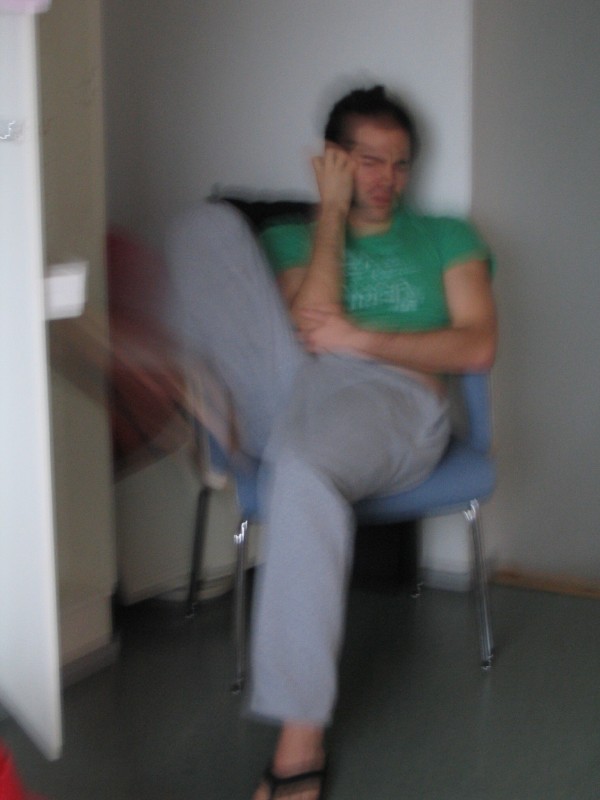In this blurry image, a man is seated in a compact room with white walls, positioned snugly into a corner. He occupies a chair with a blue cushioned seat, blue armrests, and a blue backrest, supported by four metal legs. The floor beneath him is gray in color. The man is dressed in gray sweatpants and black thong-style flip-flops; his left foot is planted firmly on the floor. His right leg is bent, with his knee drawn up towards his body, resting on the chair. He is wearing a green shirt and has his left arm folded across his stomach while his right hand is either touching his cheek or scratching his face. The expression on his face suggests that he is grimacing, indicating discomfort.